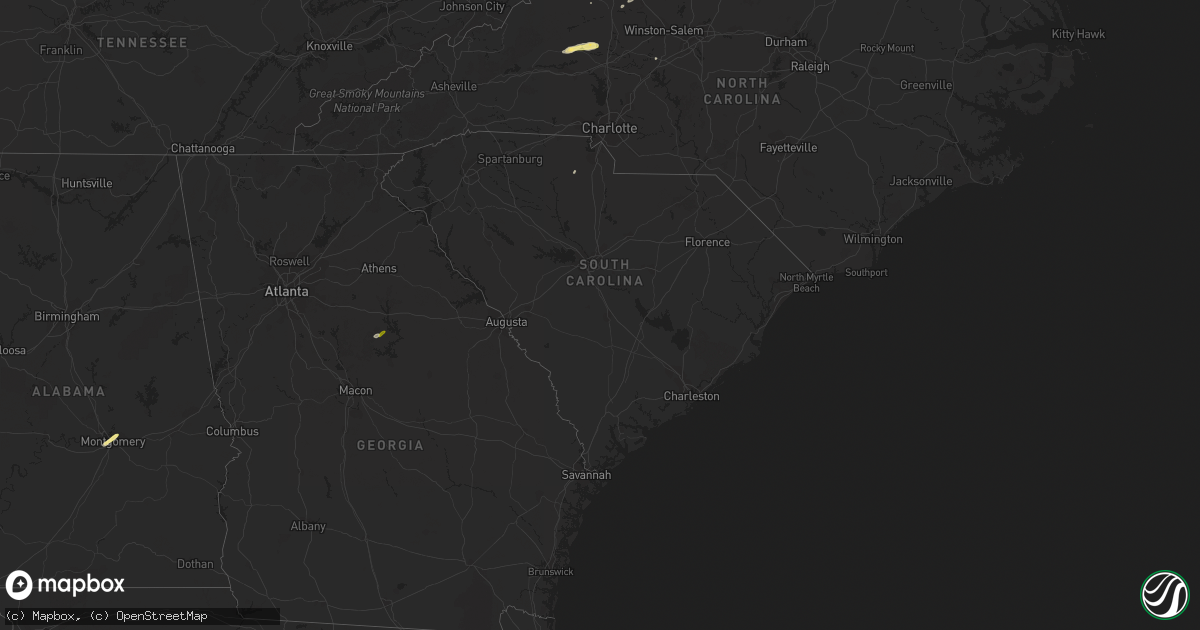A dark, radar-like map displays the southeastern region of the United States, labeled "Mapbox" at the bottom. The map extends from Tennessee in the top left corner to North Carolina, South Carolina, Georgia, and Alabama. The surrounding waters are completely black, matching the overall dark theme of the map. State names and some town names appear in dark gray text, blending into the black background and making them challenging to read. Three small, scattered orange specks likely indicate radar activity: one near Winston-Salem in North Carolina, one somewhere in Georgia (potentially mistaken for Atlanta), and another near Montgomery in Alabama. The map is titled "Open Screen Map" at the bottom.